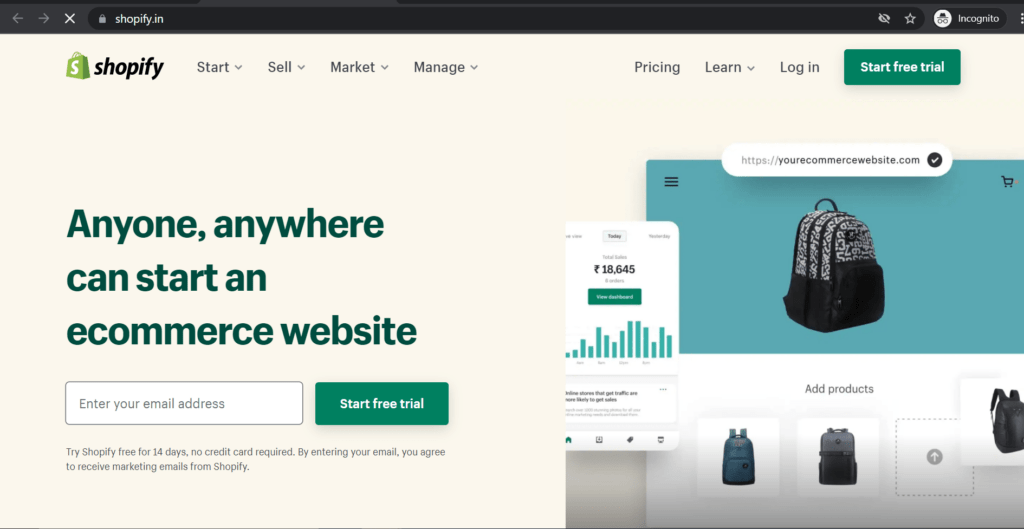This image depicts the Shopify website, specifically its Indian version, as indicated by the URL "shopify.in" visible in the browser's URL bar at the top. The upper left-hand corner of the webpage features the Shopify logo—a green, diagonally-facing shopping bag with a white "S" in the middle, accompanied by the word "Shopify" in italicized, blocky black letters.

To the right of the logo, a navigation menu appears with items in black or medium gray lettering that read "Start," "Sell," "Market," and "Manage," each accompanied by a downward arrowhead signifying drop-down menus. Further right, additional menu options "Pricing," "Learn," and "Log In" are displayed, where only "Learn" has a downward arrowhead for an expandable menu. Next to these options is a dark green rectangular button with bold white text that reads "Start Free Trial."

The main section of the website features a light beige background. Positioned towards the middle left is a bold statement in a grayish dark green font: "Anyone, anywhere can start an e-commerce website." Below this statement is an input field—a white rectangle bordered in light gray with gray text prompting users to "Enter your email address." Adjacent to this input field is another rectangular, rounded button that matches the earlier "Start Free Trial" button with white text set against a dark green background.

This detailed description of the Shopify homepage highlights its user-friendly navigation and inviting call-to-action elements designed to encourage users to start their e-commerce journey.